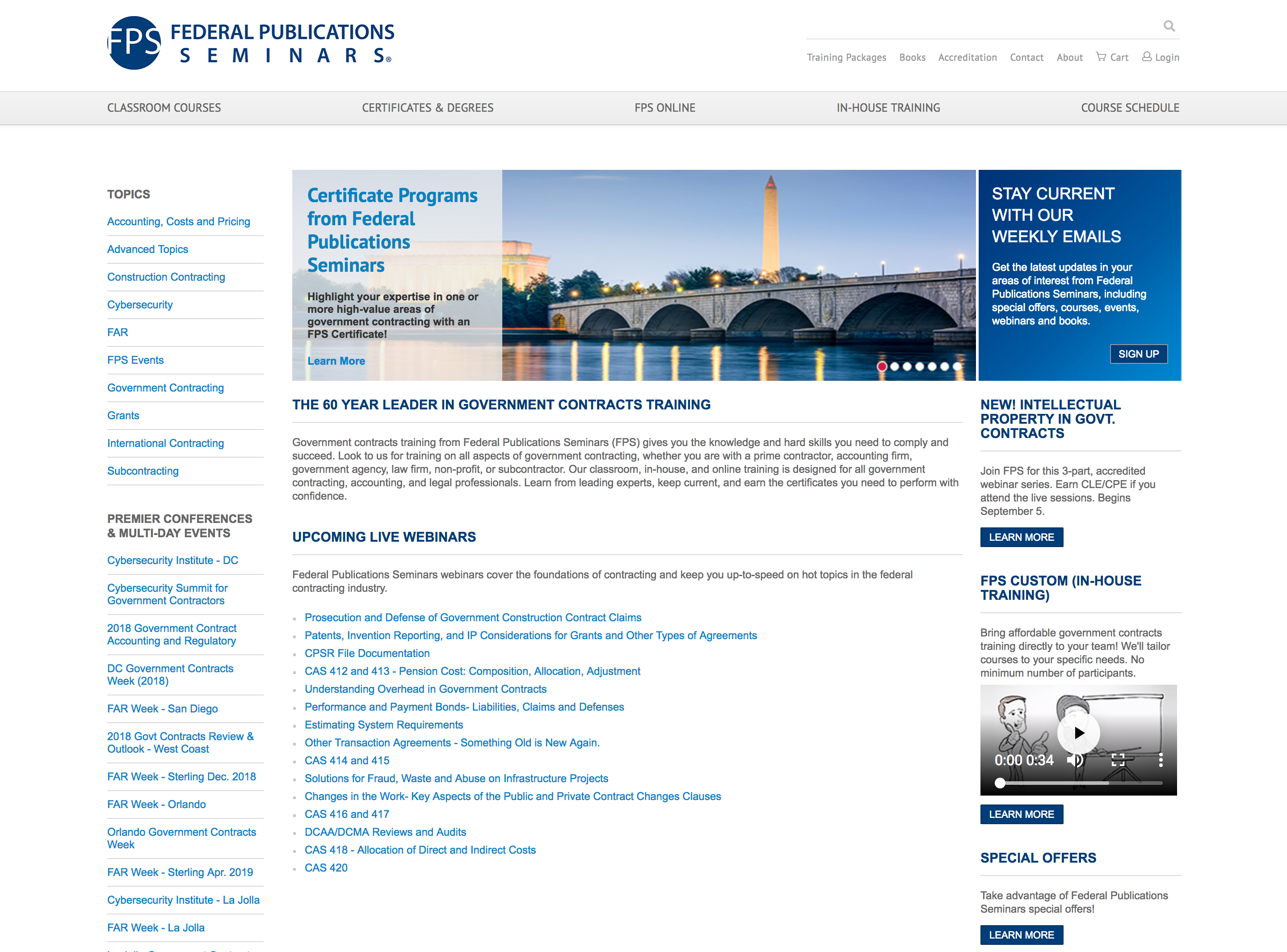The image depicts a detailed screenshot of a web page from Federal Publications Seminars. The page lacks a visible web address but prominently features the branding "Federal Publications Seminars," accompanied by a blue circle with the initials "FPS" inside.

At the top right corner, a search bar is positioned for ease of navigation, surrounded by various menu options such as Training Packages, Contact, About, Cart, Login, Books, and Accreditation. A horizontal gray bar underneath this area offers selectable options including Classroom Courses, Certificates and Degrees, FPS Online, In-House Training, and Course Schedule.

Dominating the central segment of the header, an evocative image portrays the Washington Monument illuminated against the hues of either twilight or sunrise, with the Potomac River and a bridge with multiple arches in the foreground. The Lincoln Memorial is also faintly visible, lit up but partially obscured by overlaying text. This text announces, "Certificate Programs from Federal Publications Seminars," encouraging viewers to highlight their expertise in government contracting through FPS certification, with options to learn more or sign up via a conspicuous blue button.

Further down, the site claims its status as a 60-year leader in government contracts training. It offers detailed information targeted at various types of professionals, such as prime contractors, accounting firms, government agencies, nonprofits, and subcontractors. Below this, a list of upcoming live webinars is displayed, each one highlighted in blue, suggesting clickable links.

The left-hand side of the page features a column brimming with numerous topics, along with premier conferences and multi-day events. On the right side, highlights include new intellectual property and government contracts topics, FPS custom in-house training with a currently paused video, and a section on bring affordable government contracts training directly to teams. There are also special offers for visitors to take advantage of Federal Publications Seminars' services. The page is not annotated or highlighted in any way, presenting a clear and comprehensive screenshot of the website.